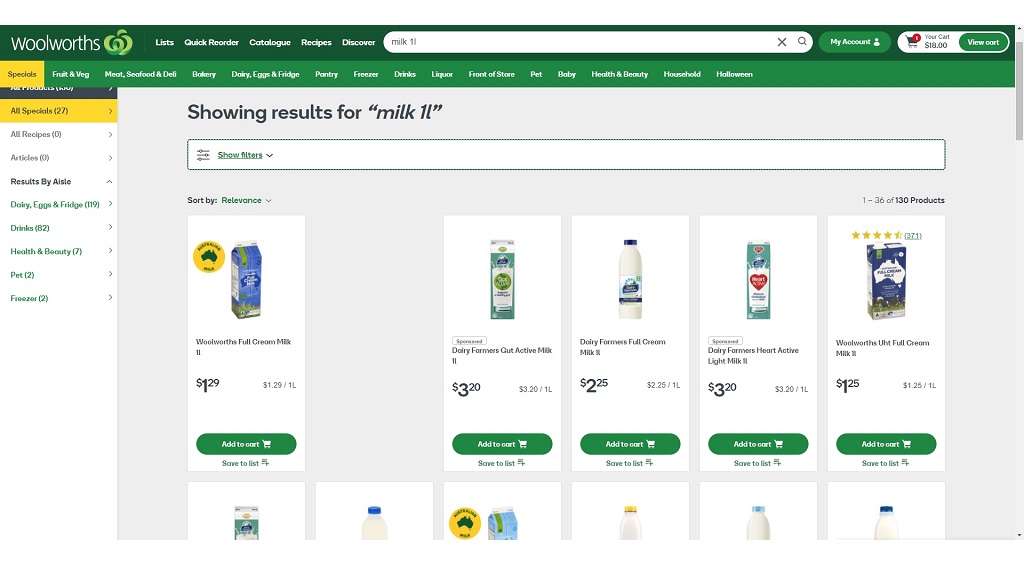The image showcases the Woolworths website displaying search results for “milk 1L.” At the top, the Woolworths logo appears with "Woolworths" in white text, in lowercase except for the capital "W," accompanied by the iconic swirly green "W" logo. To the right, navigation options include "Lists," "Quick Reorder," "Catalog," "Recipes," and "Discover." The search term entered is “milk 1L 1 liter.” Further options include "My Account" and "Your Cart."

Beneath this, the main menu categories are listed: "Specials," "Fruit & Veg," "Meat, Seafood & Deli," "Bakery," "Dairy, Eggs & Fridge," "Pantry," "Freezer," "Drinks," "Liquor," "Front of Store," "Pet," "Baby," "Health & Beauty," "Household," and "Halloween." Each of these is clickable.

To the left, a sidebar provides filtered results showing:
- All Specials (27)
- All Recipes (0)
- Articles (0)
- Result by Aisle:
  - Dairy, Eggs & Fridge (119)
  - Drinks (82)
  - Health & Beauty (7)
  - Pet (2)
  - Freezer (2)

In the center, the search results for “milk 1 liter” are displayed. Users have the option to filter and sort the results by relevance. Featured products include:

1. **Woolworths Full Cream Milk (1 liter)**
   - Price: $1.29
   - "Add to Cart" button in green with white text
   - Option to save to a list

2. **Dairy Farmers Gut Active Milk (1 liter)**
   - Price: $3.20
   - "Add to Cart" button in green with white text
   - Option to save to a list

3. **Dairy Farmers Full Cream Milk (1 liter)**
   - Price: $2.25
   - "Add to Cart" button in green with white text
   - Option to save to a list

4. **Dairy Farmers Heart Active Light Milk (1 liter)**
   - Price: $3.20
   - "Add to Cart" button in green with white text
   - Option to save to a list

5. **Woolworths UHT Full Cream Milk (1 liter)**
   - Price: $1.25
   - Rating: 4.5 stars from 327 reviews
   - "Add to Cart" button in green with white text
   - Option to save to a list

Each product listing includes a thumbnail image of the milk carton above the product details. Below these primary listings, there are six additional preview images of other milk cartons, though only the top portion is visible.